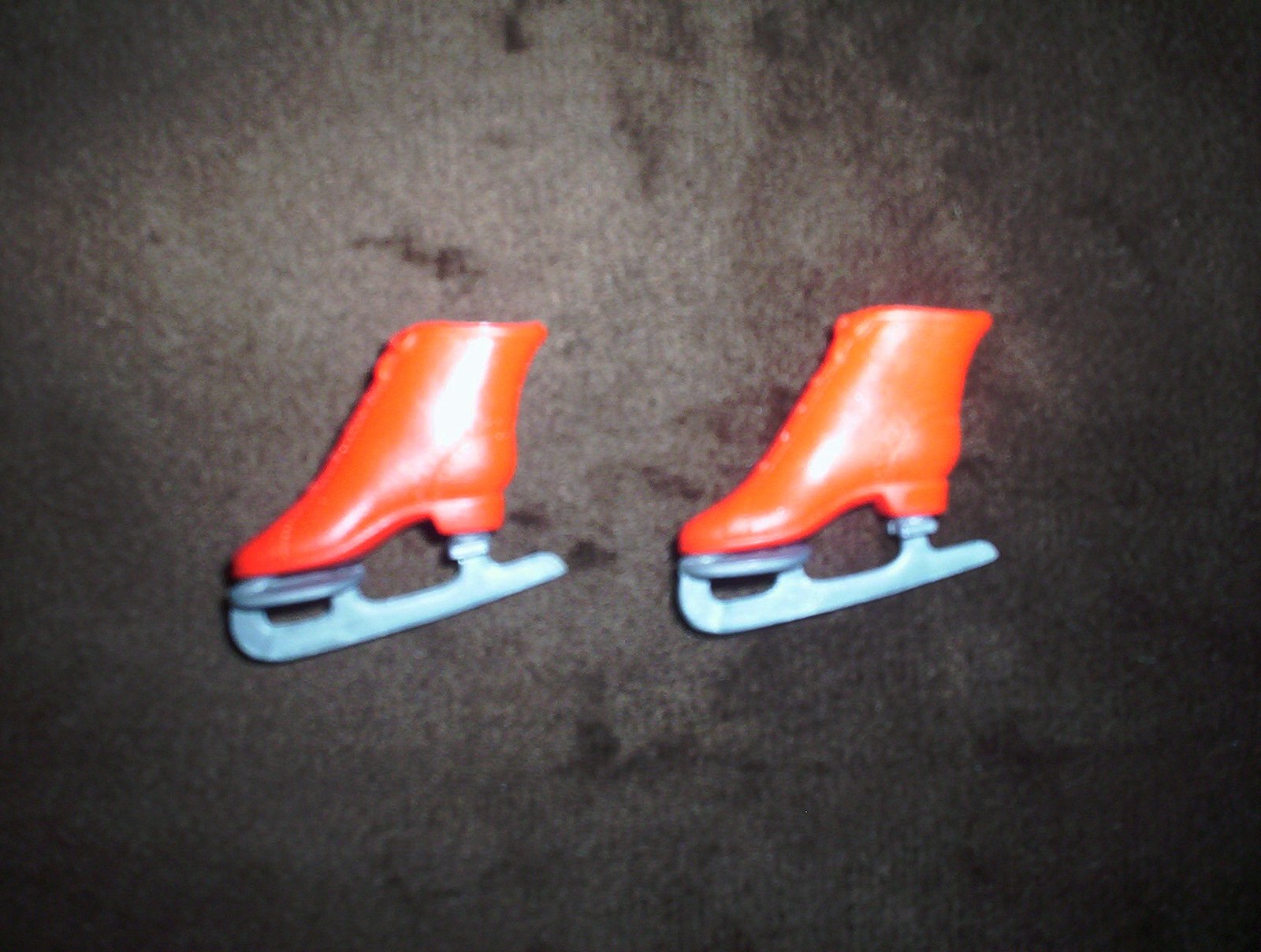The image displays a pair of small, plastic ice skates designed for dolls, with bright red-orange boots and blue-silver painted blades. The boots, which are high-heeled and appear to lack strings, are positioned side by side, facing left. The skates, likely reflecting camera flash, rest on a dark brown carpet that is lighter in the center where the skates lie, creating a spotlight effect. The background features subtle creases and darker areas towards its edges, giving it a slightly textured appearance. Despite looking shiny, the skates appear to be toy-like and not very well-constructed.